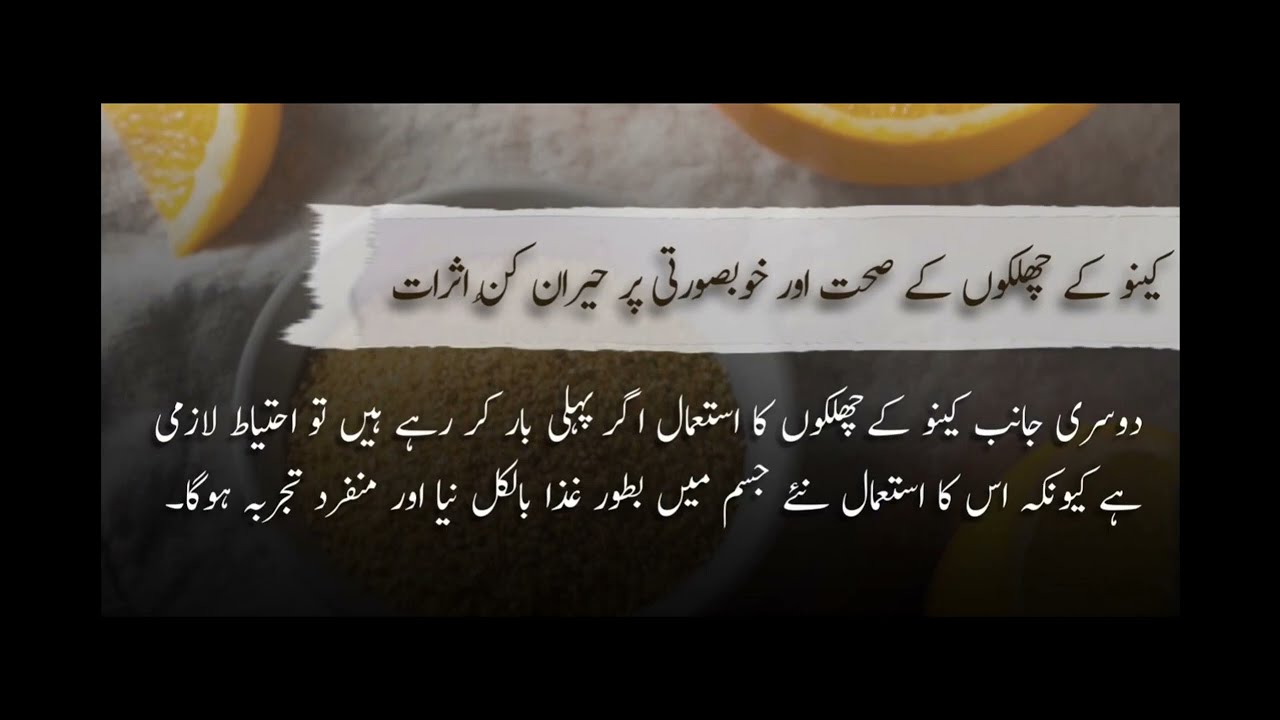The image is a graphical design with a thick black rectangular border and a horizontal orientation. The black background has a wider bottom section that gradually fades into the picture, while the other edges are sharp. Within this border is a dimmed, close-up graphical depiction of a table scene featuring slices of oranges and what seems to be a white bowl containing a tan-colored, crumbly substance, possibly couscous or spices. The top of the graphic slightly crops the lemon wedges. Across the middle of the image runs a white, paintbrush-stroke-like rectangle with dark Arabic text, adding a naturalistic effect. Beneath this painted banner, on the black gradient overlay, are two lines of white Arabic text.